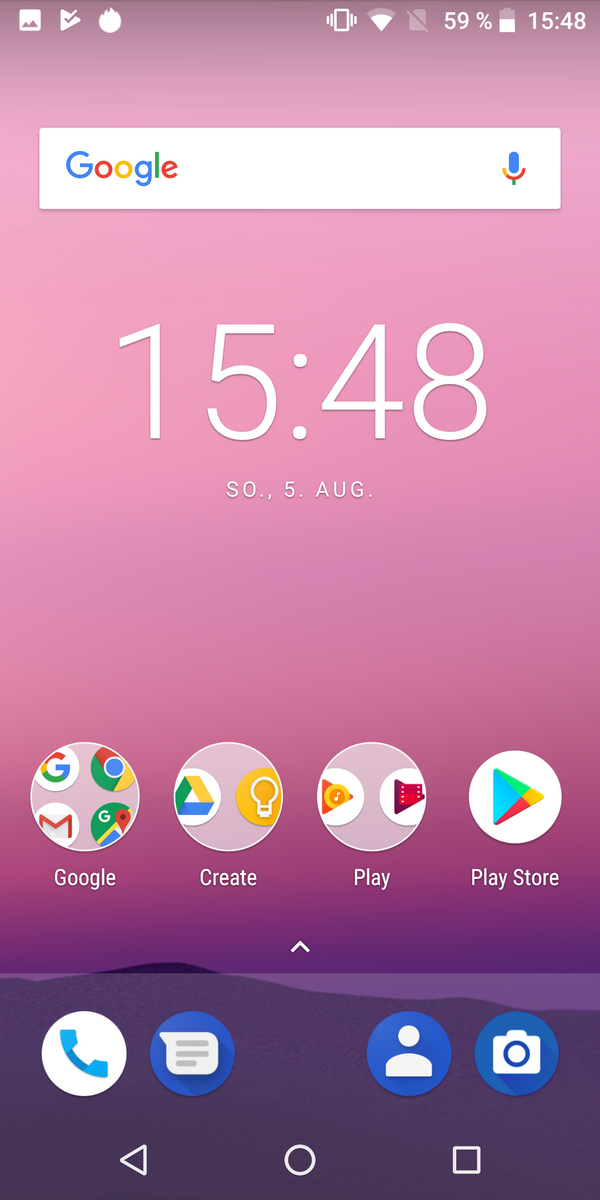This image showcases the homepage of a mobile device, likely a smartphone, capturing a user's personalized interface. The background gradient transitions from a mauve shade at the top, through a purplish hue in the middle, to a deeper purple, almost black, at the bottom.

At the top of the screen, prominent against the soft mauve, is the iconic multi-colored "Google" logo situated within a search bar. Adjacent to this is a white space, which houses a blue-tipped microphone icon for voice searches.

Central to the image is a large digital clock displaying "15:48." Just below the time, the text indicates the date with a format of "Sun, 5 Aug," aligning left and blending harmoniously with the overall background gradient.

Towards the bottom, various circular app shortcuts are visible, including icons labeled "Google," "Create," "Play," and "Play Store." Beneath these, set against the darkest segment of the gradient, are additional icons representing essential functions: a phone, a text message bubble, a human silhouette (most likely for contacts), and a camera icon. This detailed description captures the structured and user-friendly design of a customized mobile device homepage.